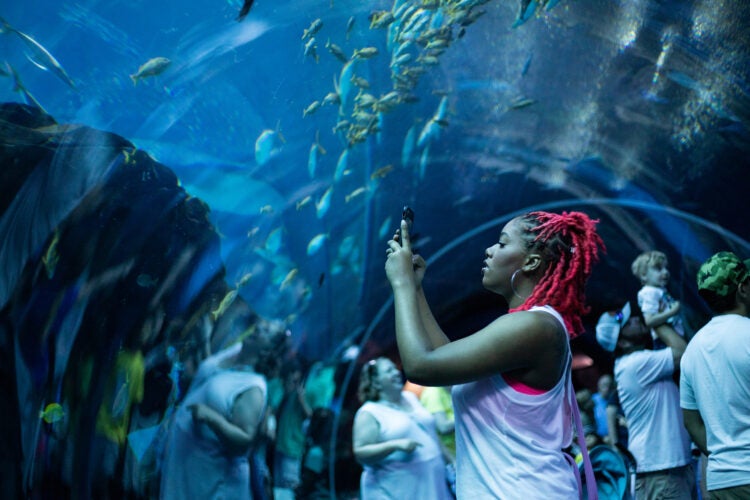This photograph captures the captivating scene of an underwater tunnel aquarium. The tunnel is semi-circular in shape, constructed with transparent glass walls that immerse visitors in the aquatic environment. Inside the tunnel, there are roughly ten people standing and gazing at the mesmerizing marine life. Closest to the viewer is a black woman with red dreadlocks tied back, wearing a white top. She holds her phone aloft, likely capturing the enchanting sight around her. Above and around the tunnel, a school of small green and yellowish fish, about 20 to 30 in number, swims gracefully in the blue-hued water. Among the crowd, a man is seen holding up a child to give them a better view of the aquatic display. Reflections on the glass add an intriguing layer to the image, blending the spectators' silhouettes with the vibrant marine life, enhancing the sense of being truly submerged in the ocean's wonders.